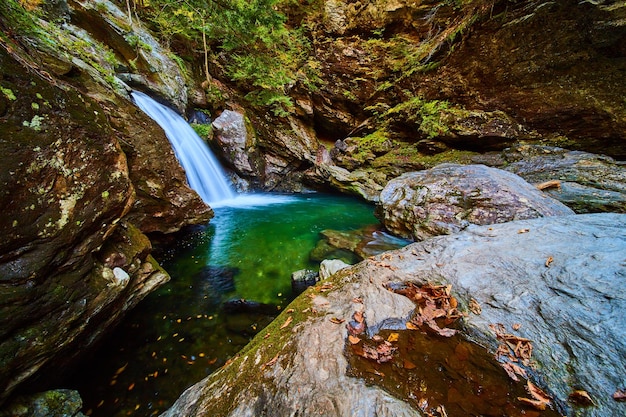This detailed image captures a serene natural scene set in a deep, steep ravine. A small waterfall cascades from the left, feeding into a clear, light green pool dotted with floating leaves. The stream flows gently to the left, surrounded by various rocks and vegetation. To the bottom right, large gray stones are strewn with dead leaves. The top right features brownish stones adorned with patches of green moss, small plants, and bits of grass, adding a touch of vibrant life to the rocky landscape. Just in front, a prominent gray rock with a puddle reflecting a brownish hue sits, partially covered with dark green moss. Over on the left side, tree leaves frame the scene, adding greenery above the cascading white falls. The entire image suggests a lush, forested environment, epitomizing the tranquil beauty of nature.